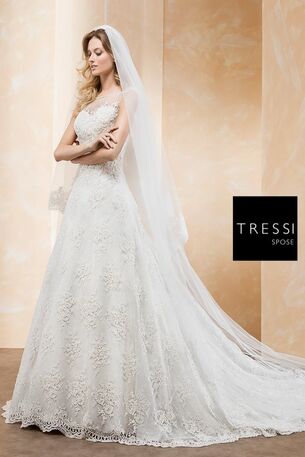In an indoor setting, a fair-skinned bride stands gracefully in the center of the image, her arms gently crossed and her gaze directed downward. She has brown, wavy hair cascading down to her upper arms, and she wears a white, sleeveless wedding dress. The dress is adorned with intricate lace patterns, floral motifs, and a sheer cover extending to her leg area, finishing with a delicate lace edge at the bottom. Her outfit includes a trailing wedding veil that complements the dress's elegance. The background features a series of beige panels with vertical lines, enhancing the bridal attire's pristine white color. To the right side of the image, there is a black square displaying the text "TRESSI" in bold white letters, followed by "SPOSE" in a smaller font below. The setting suggests either a wedding ceremony or a staged photoshoot, with a color palette including white, tan, brown, a hint of pink, and gray, with the floor possibly being a gray carpet.